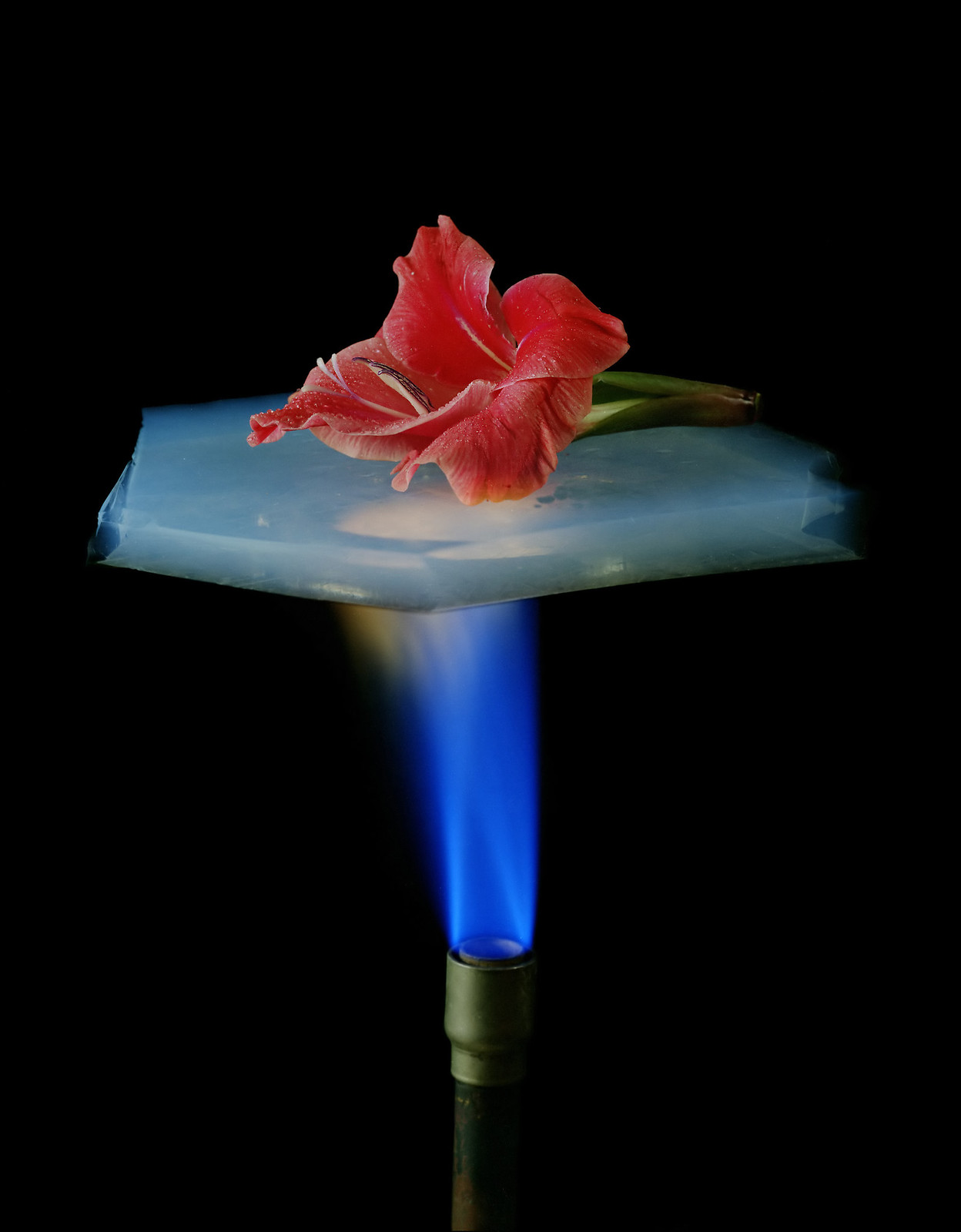This image depicts an intricate and surreal scene set against a stark black background. At the center of the composition is a striking tropical flower, which appears to be a bird of paradise, characterized by its bold reddish-orange petals and green bud. The flower is perched delicately on a translucent glass prism, which exhibits multiple layers and has a light blue hue reminiscent of marble or slate. Below the prism, a blue flame, emitted from a burner with a green nozzle and a rusted pipe, creates an ethereal effect by interacting with the glass, resulting in yellow tinges at the flame's top. The combination of the vibrant red and orange petals, the prismatic glass, and the hypnotic blue flame lends the image a fantastical quality, capturing a moment where nature and science fiction converge in a visually captivating and unexplained phenomenon.